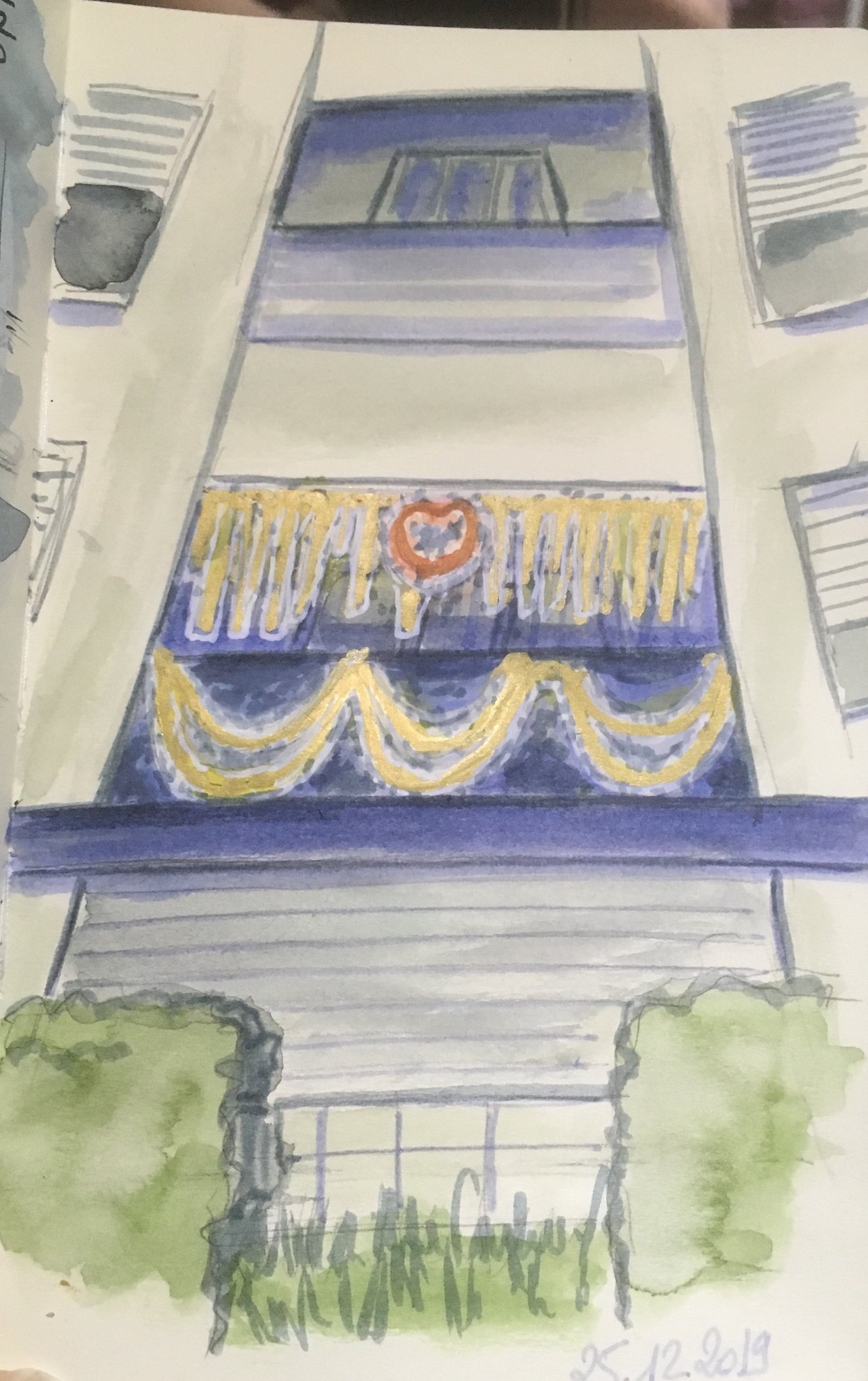The image depicts a muted, pastel watercolor painting of a minimalist, multi-story building against a white background. The artist has signed it "K.12.2019" in the bottom right-hand corner. The foreground features green bushes and trees, with hints of a figurine standing beside one tree on the left and additional greenery on the right. At the base of the building, there appears to be a gray garage door. Moving upwards, the building showcases a series of windows outlined in gray, with distinctive blue accents. The first level features a blue section decorated with yellow banners and a red heart. Above, there's another patio in different shades of blue and white, adorned with vertical gray lines. Overall, the composition combines simplistic architectural elements with subtle, earthy tones, creating a serene and cohesive scene.